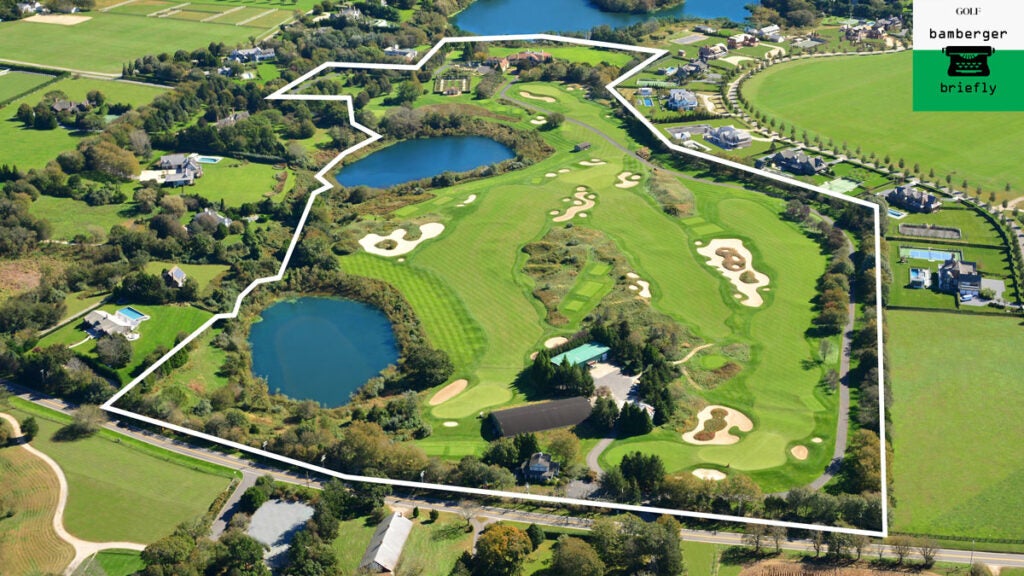This aerial photograph captures a lush, green golf course delineated by a white border showcasing its boundaries. The meticulously manicured fairways and greens are interspersed with multiple sand traps of varying sizes, giving the course a textured and patterned appearance. There are three bodies of water within the course: two small ponds nestled within the golf course boundaries and an additional pond at the upper edge, just outside the white border. The course is surrounded by various shrubs and trees, adding to its scenic beauty.

Encircling the golf course are several residential properties, many of which feature swimming pools in their backyards. Rows of homes can be seen particularly on the right-hand and left-hand sides of the image. In the back left of the shot, a tennis court is visible, adding to the recreational amenities in the area. At the bottom edge of the photograph, a road runs diagonally from left to right, marking the forefront of the golf course. Adjacent to this road are a couple of structures that appear to be country club buildings. An old-fashioned typewriter label "Golf Bamberger" can be spotted in the upper right corner of the image, adding a distinctive touch to the overall scene.